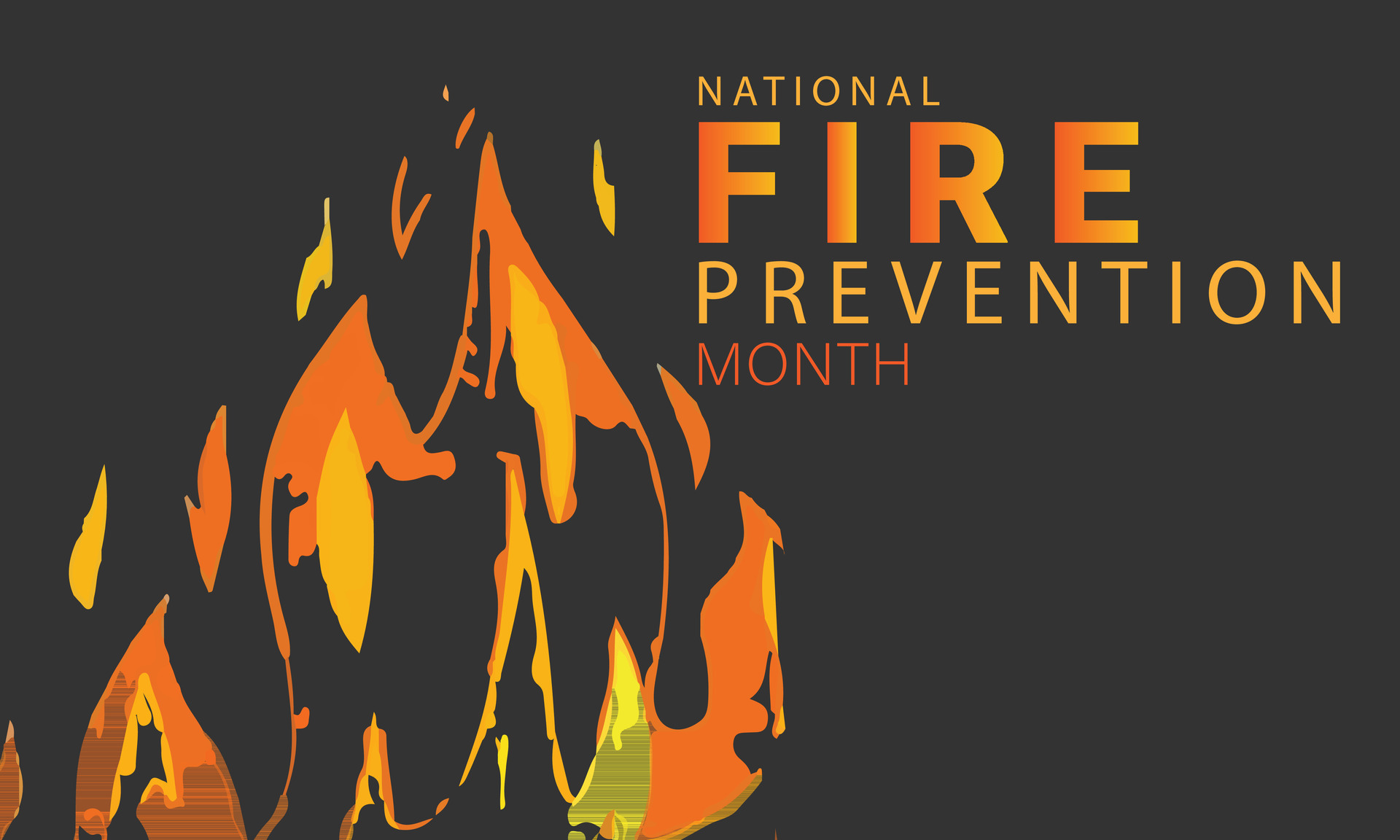This image is a graphic poster for National Fire Prevention Month. The background is predominantly a dark gunmetal gray, giving it a stark and dramatic tone. On the left side of the image, from the bottom to almost the top, there's a stylized image of a flame, primarily outlined in orange with intricate yellow details. This flame appears to be semi-translucent, revealing faint silhouettes of buildings or other structures through its base.

Positioned on the upper center to the right-hand side of the image, the text reads "National Fire Prevention Month." The word "Fire" is the largest, rendered in a striking gradient of orange to yellow. "National" and "Prevention" are in vivid yellow, and "Month" is highlighted in a strong orange hue. The varying shades of orange and yellow in the text complement the colors used in the flame illustration, creating a cohesive and visually impactful layout.